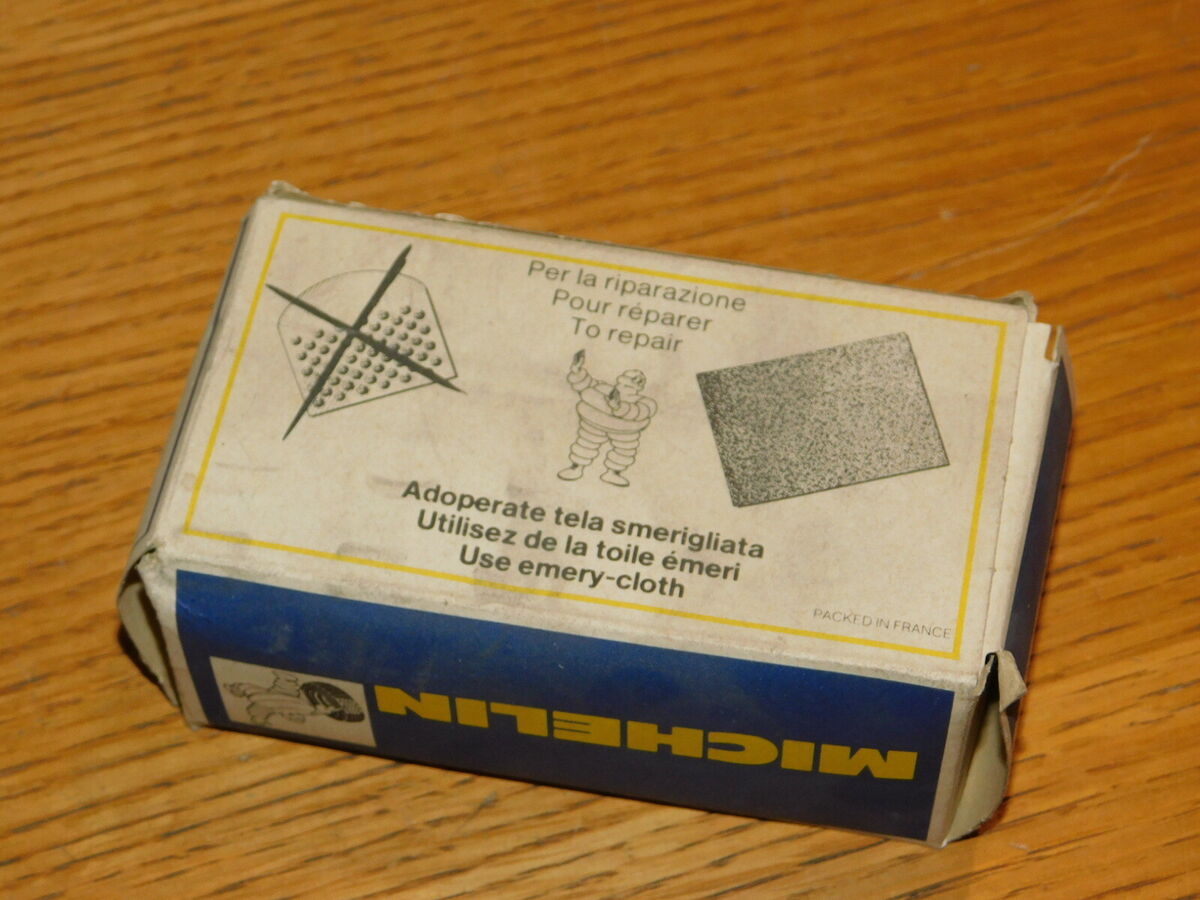The photo depicts a vintage blue and white Michelin box placed on a wooden desk. The box, which shows signs of wear and tear, likely dates back to the 1960s or 1970s. Prominently featured on the box is the iconic Michelin Man, a white, marshmallow-like character made to appear as if assembled from tires. The Michelin Man logo appears both in an illustration on the front and on the side of the box, against a blue background with yellow lettering.

The text on the box includes instructions in multiple languages, with English instructions stating "To Repair, Use Emery-cloth." The packaging, proudly marked as packed in France, also contains some unreadable French text on the back. The back of the box features illustrations, one of which shows a crossed-out image of a cloth, possibly indicating that it should not be used, while another illustration depicts the approved emery-cloth. The Michelin Man is seen in a rejecting pose towards the crossed-out cloth illustration, while appearing approving towards the correct emery-cloth illustration.

Overall, the image seems to capture the photographer's intent to showcase this intriguing historical find.